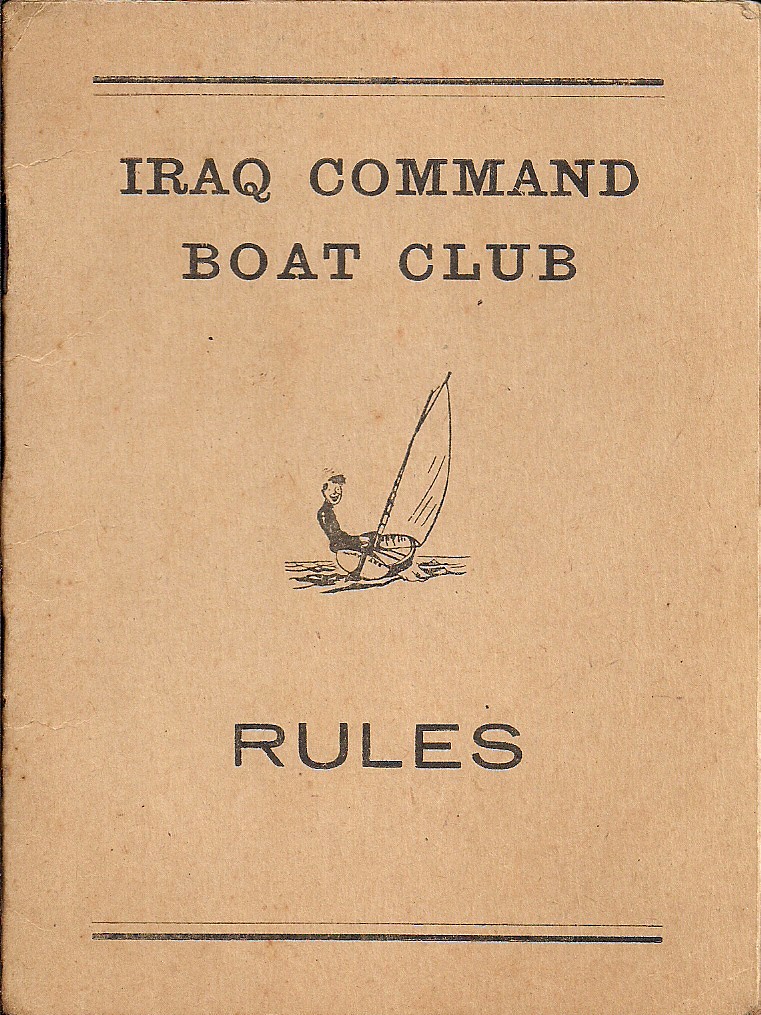The image is a scanned cover of a rule book for the "Iraq Command Boat Club." The cover is colored in a light tan, resembling a brown paper bag or woodgrain texture. At the top, a thick black line runs almost edge-to-edge, followed by a thinner black line beneath it. Below the lines, the title "IRAQ COMMAND BOAT CLUB" is printed in capital letters. In the center of the cover, there's a cartoon-style, hand-drawn graphic showing a person in a small boat that appears to either have a fishing rod or a sail, navigating a patch of water. Underneath the illustration, the word "RULES" is prominently displayed. The bottom of the cover features another thick black line, mirroring the top design. The cover's sides reveal the potential presence of two or three staples along the left border.